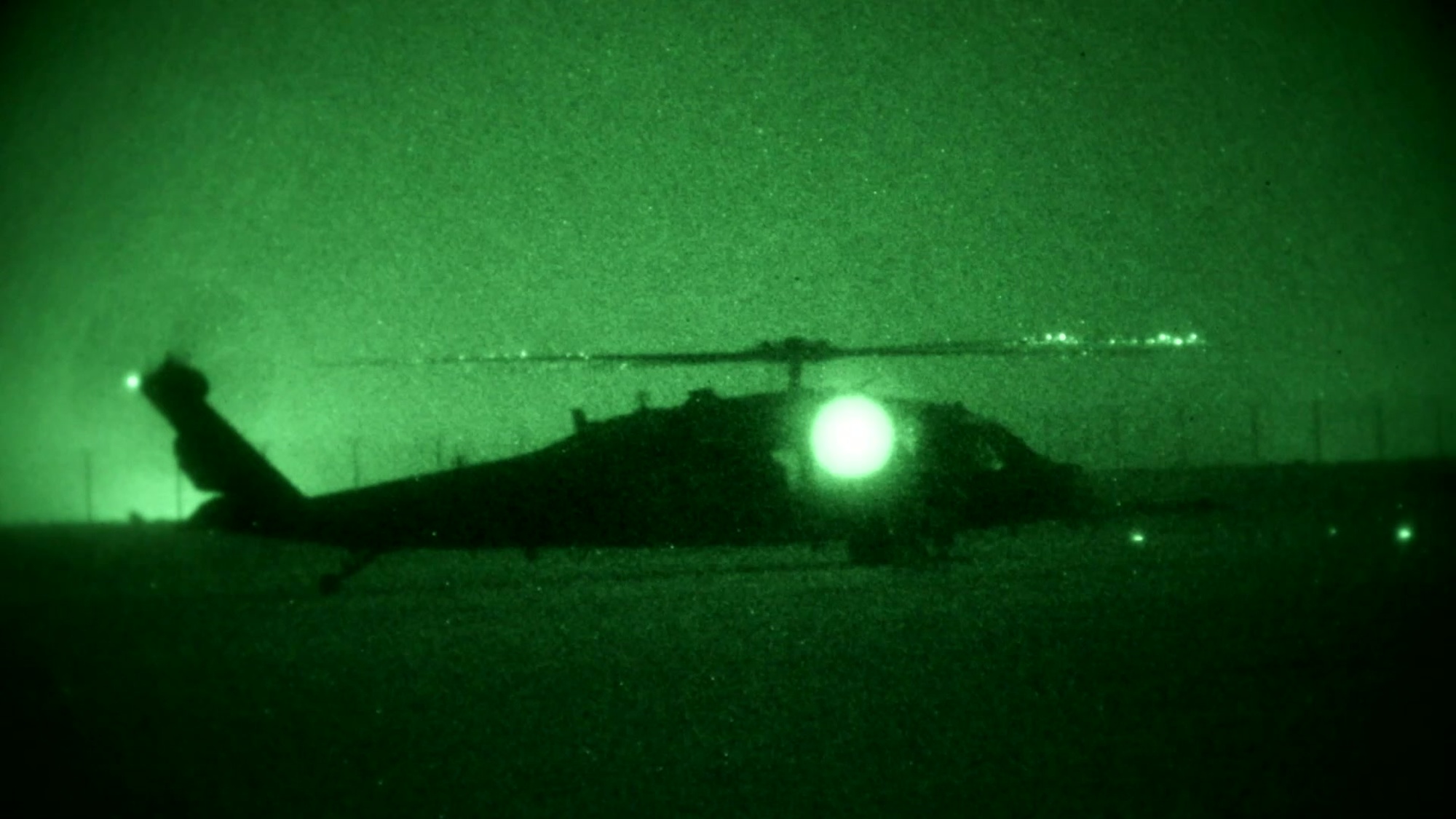In this night vision photograph, a military helicopter is captured from the right side, bathed in the characteristic green hue of night-vision technology. The helicopter's main blades and tail rotor are visibly spinning, suggesting it is operational. A bright light reflects prominently off the cockpit, likely an external light source illuminating the helicopter. In the background, a series of electric poles stretches out towards the horizon, adding depth to the open field setting. A metal fence can also be seen near the base of the helicopter, indicating a restricted or secured area, possibly a military base. The green hue and prominent circular light reflection center-frame add an eerie, surreal quality to the image, accentuating its night-time military ambiance.